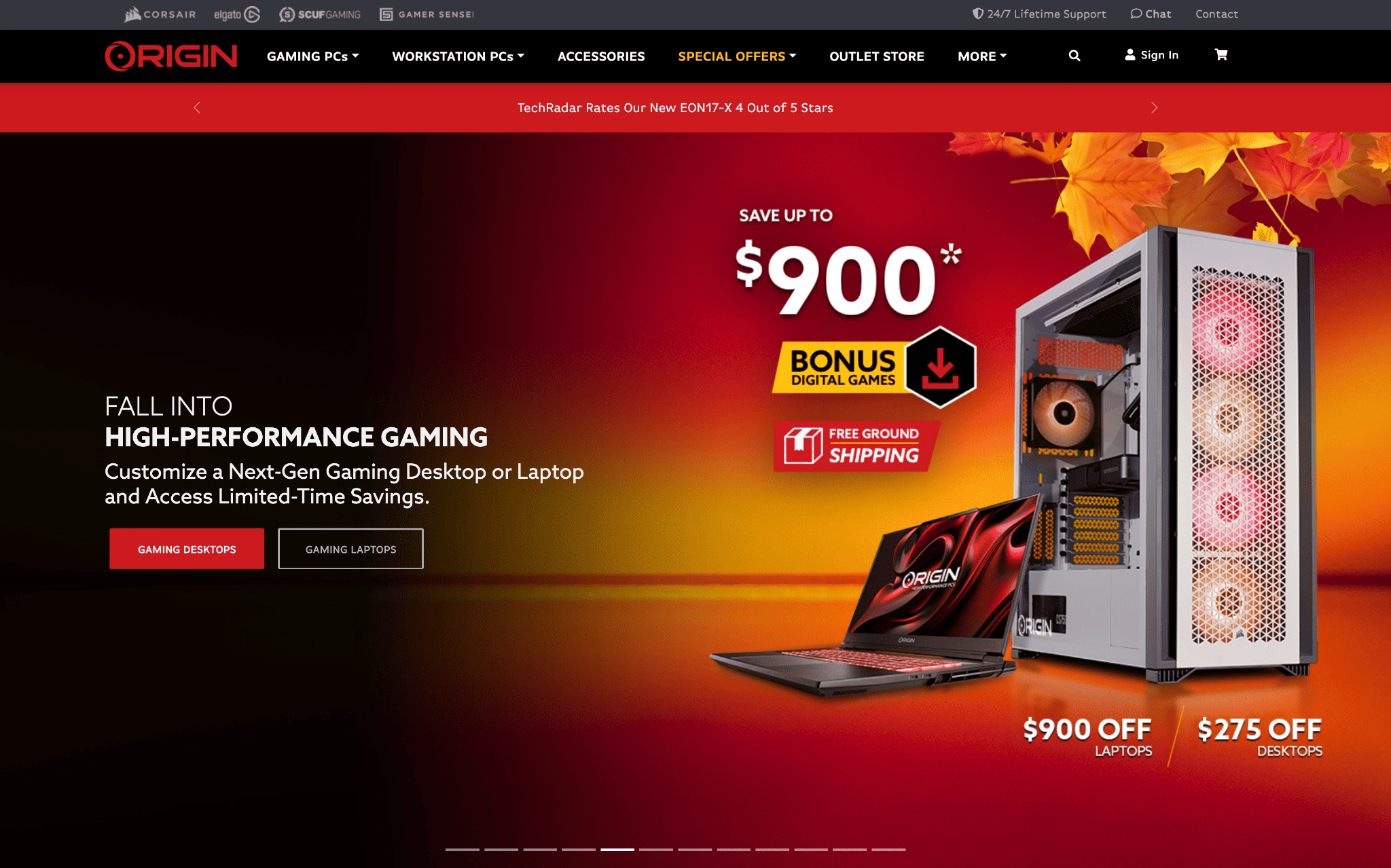Discover unbeatable deals on cutting-edge gaming systems with Origin PC. Experience high-performance gaming this fall with customizable next-gen gaming desktops and laptops, and enjoy limited-time savings. You can save up to $900 on select laptops and $275 on select desktops, both of which come with bonus digital games and free ground shipping.

Featured in this offer is a sleek gray desktop with vibrant orange LED fans illuminating the interior, providing a striking aesthetic element against the red background adorned with orange leaves. Alongside it is a sophisticated black laptop, also part of the substantial discount offerings.

Take advantage of 24/7 lifetime support, and easily reach out via chat or contact options. Don't miss out on these exceptional savings and the opportunity to enhance your gaming setup with top-of-the-line equipment from Origin PC.